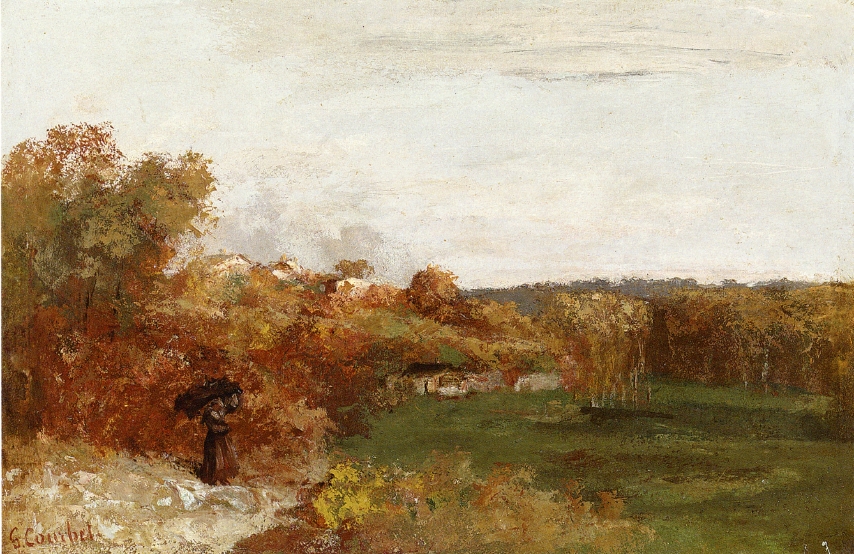This impressionist style painting captures a serene fall outdoor scene with remarkable detail and vivid colors. Dominated by a palette of greens, browns, and rust, the painting features a green grassy clearing at the center, encircled in a horseshoe shape by an array of trees with foliage in hues of red, brown, yellow, and a touch of green. The trees' trunks display splashes of white paint, adding depth to the composition. In the bottom left corner, the artist's name is inscribed. Above this signature, a shadowy figure wearing 17th-century attire, including a brown dress and holding a brown umbrella, stands prominently. The figure seems to be one of possibly two people depicted, thus providing a focal point amidst the landscape. Surrounding the clearing, the landscape morphs into a dense area filled with trees and bushes, transitioning from dark light green to rusty tan shades, further accentuated by a dimly visible hill in the background. Overarching the entire scene, a washed-out, light gray sky with darker gray clouds portrays an overcast and moody atmosphere, enhancing the autumnal theme of the painting.